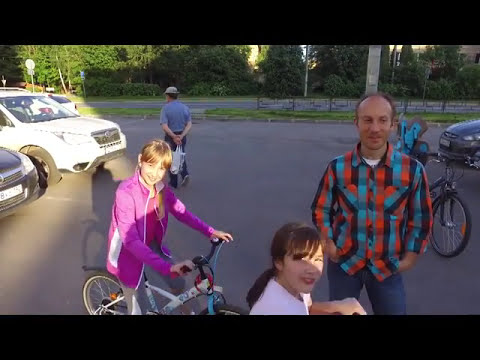The image, framed by horizontal black bars at the top and bottom, features a diverse scene with four people and several objects. Dominating the right side is an older, slightly balding man clad in a plaid shirt with black, red, and blue checks, paired with blue jeans. His hands are in his pockets, and he is smiling while gazing off to the right. Just behind him, partially visible, is a bike outfitted with a blue child carrier. In the background, on the left, another man in a white hat is walking away, hands behind his back and carrying a plastic bag; he is dressed in a blue shirt. 

In the foreground, two young girls are the primary focus. The girl on the left is in a bright pink sweater, smiling directly at the camera. She is riding a blue and white bicycle with a hint of purple on her jacket. Her companion, to the right, is wearing a white shirt; while most of her body is cropped out, the position of her hands suggests she is also on a bike. Both girls have bangs, and the sun catches the girl in white, casting half her face in light. Surrounding them is a parking lot with several cars: a black and a white car on the left, a silver one to the right, and another vehicle positioned behind the man. The road stretches across the background, from left to right, completing this lively outdoor snapshot.